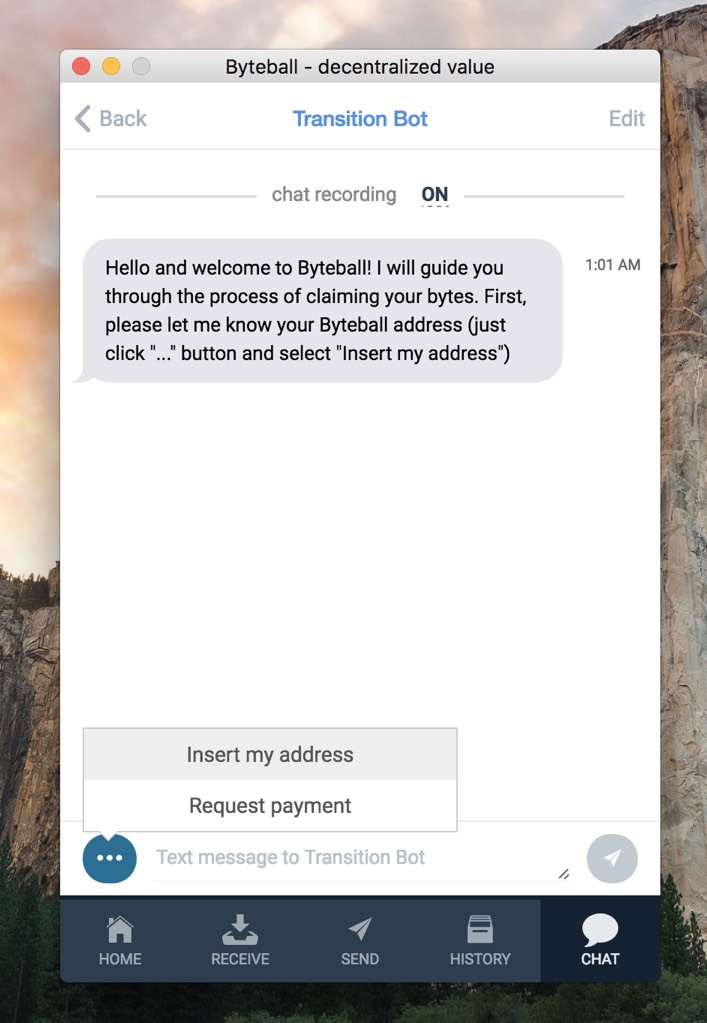The image features a busy interface obscuring a scenic outdoor screensaver in the background. The serene backdrop includes a wide expanse of sky predominantly on the left side, transitioning into a rural landscape with a mountain or hill on the right. Pine trees are discernible in the lower right corner, peeking through the interface clutter.

Dominating the scene is a large chatbox presenting a conversation with a chatbot. Across the top of this interface, the words "Byteball, Decentralized Value" are prominently displayed. To the left, a small arrow labeled "Back" offers navigation, while the center spotlights the text "Transition Bot" in blue. On the far right, the word "Edit" is visible. Below this header, instructions are given for the chat with "Chat Recording: ON" noted in capitals.

The chatbot text reads, "Hello and welcome to Byteball. I will guide you through the process of claiming your bytes. First, please let me know your Byteball address. Just click '...' button and select Insert my address." To the right, the timestamp shows "1:01 AM".

At the bottom of the interface, two option buttons are present: "Insert My Address" with a gray background and "Request Payment" with a white background. Additionally, a navigation bar at the very bottom provides icons labeled Home, Receive, Send, History, and Chat.